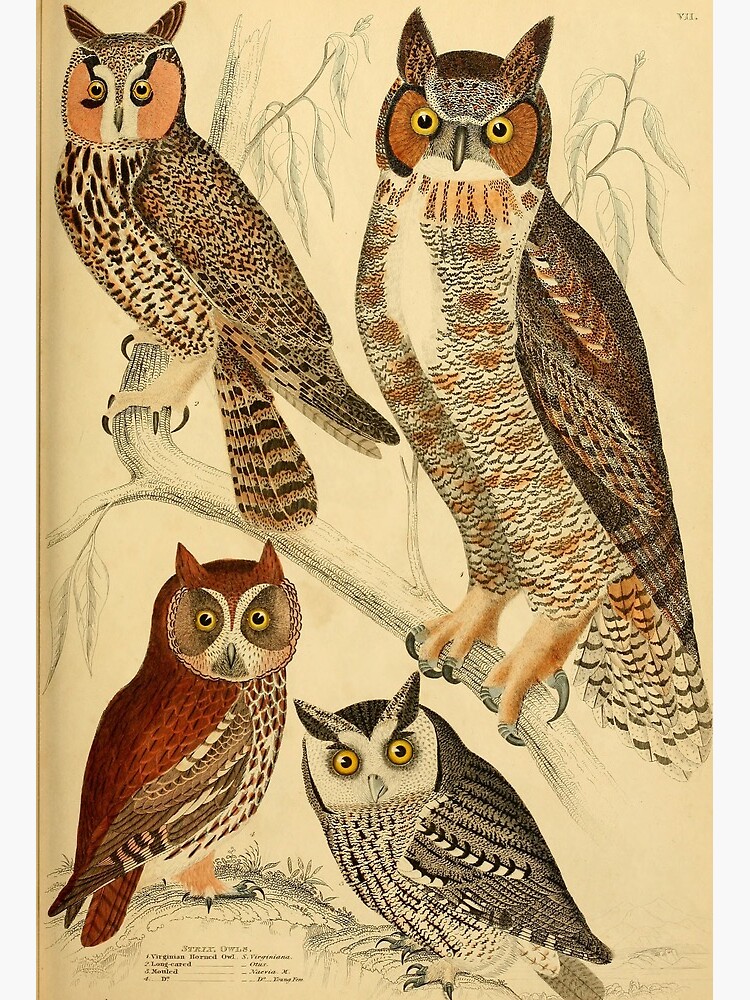The image depicts a meticulously drawn scene featuring four owls on a beige background. The illustration combines a pencil background with earth-toned colors, primarily muted browns, oranges, yellows, and blacks, bringing depth and character to the owls. Two larger owls, adorned in brown and gold hues, perch prominently on a detailed branch, staring intently with their large yellow eyes. These owls, positioned front and center, exude a commanding presence. A smaller reddish-brown owl perches alone at the bottom left, its vibrant red tones and distinctive beak adding a striking contrast. Adjacent to it, a darker brown owl with pronounced, sharp feather tufts above its eyes shares the scene. This owl also features an orange face with a lighter orange area on the front, contributing to the diverse coloration of the group. The background resembles pencil-drawn textures on beige paper, while the owls are colored with precision, making the drawing appear both antique and detailed. There's some text at the bottom of the image, but it's too small to read. The overall composition, with its natural hues and intricate details, is evocative of an old tapestry or a fine painting, perfect for framing and display.